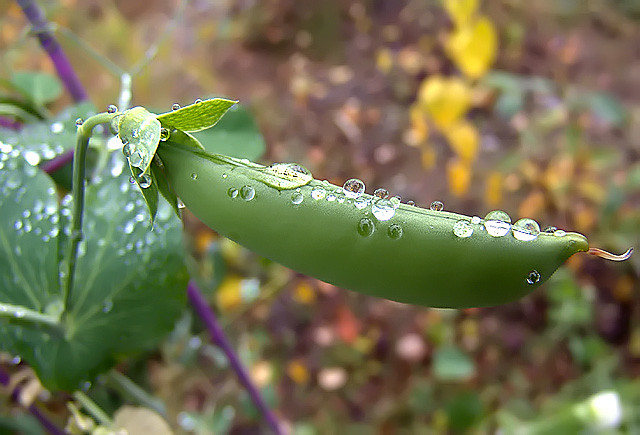In this realistic outdoor image, the central focus is a vibrant green peapod adorned with large dew drops, making it appear freshly kissed by rain. The peapod has a straight appearance with a curly tail extending to the right. Behind the peapod, the background is artistically blurred, featuring hints of various vegetation including splotches of yellow, red, and green, potentially flowers or leaves, contributing to an impression of a garden or forest-like setting. A notable feature in the composition is a heart-shaped, glistening green leaf to the left of the peapod, also dotted with water droplets. Additionally, two parallel purple stalks emerge diagonally in the frame, enhancing the natural beauty of the scene. The overall image exudes a lush, vibrant atmosphere, suggestive of a post-rainfall garden.